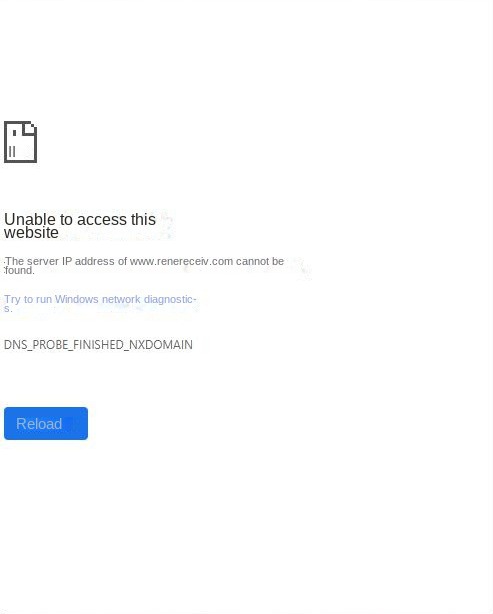The image depicts a white web page displaying an error message indicating the inability to access a website. At the top, there is an icon resembling a tilted letter, followed by a prominent headline in black text stating "Unable to access this website." Below this, another line of black text reads "The server IP address of www.runnerreceive.com cannot be found." Further down, there is a clickable blue link in white text that suggests, "Try to run Windows Network Diagnostics." The subsequent line of text, also in black and in all uppercase, displays "DNS_PROBE_FINISHED_NXDOMAIN." At the very bottom of the page, there is a blue button with white text that says "Reload." The entire page has a plain white background with all the text in black, except for the blue link suggesting network diagnostics and the blue reload button at the bottom.